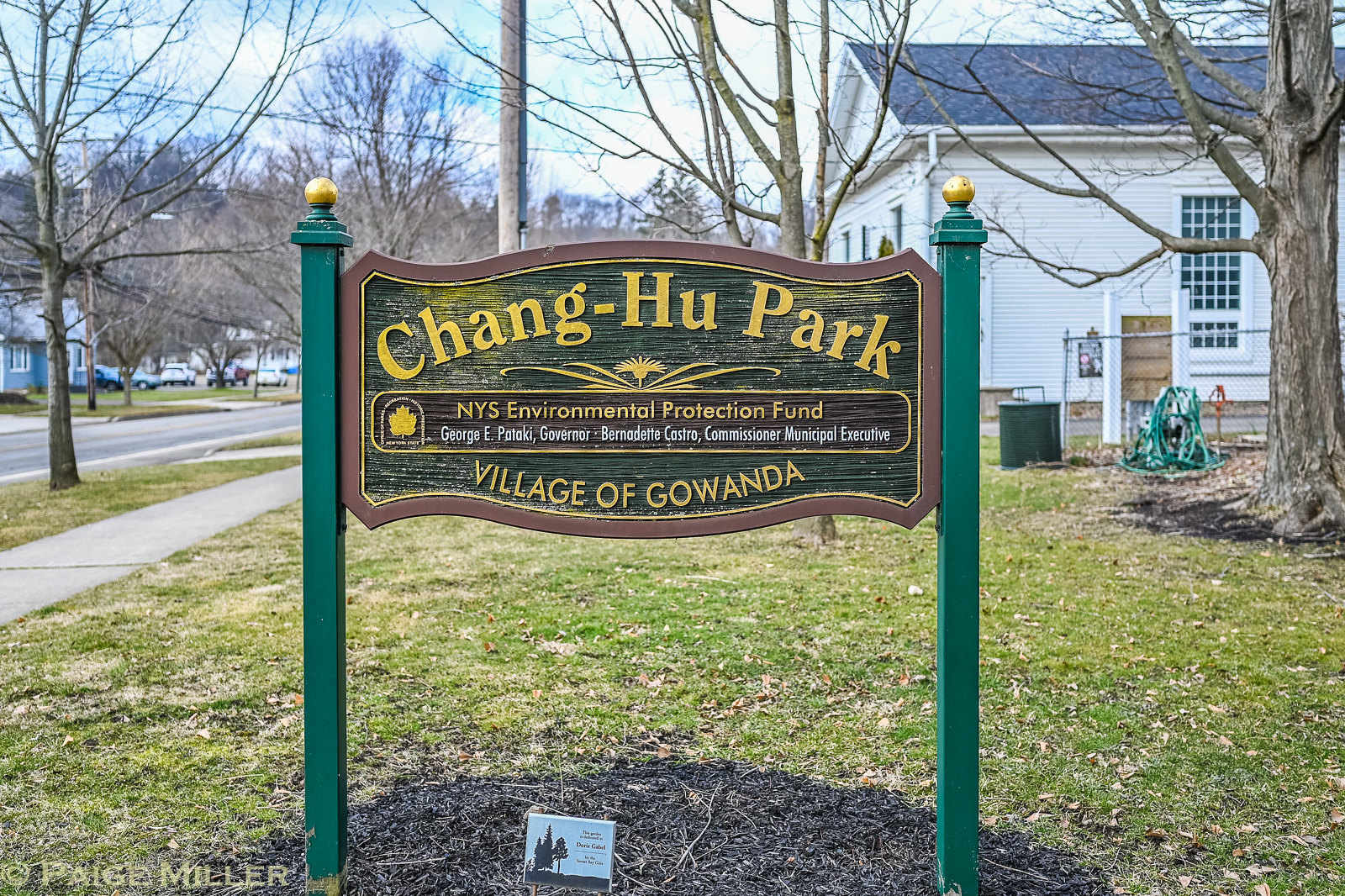In the image, a prominently positioned wooden sign stands front and center, flanked by two green poles and anchored in a grassy area interspersed with patches of mulch and dead leaves. The sign reads, "Changhu Park, NYS Environmental Protection Fund," listing figures such as George E. Pataki, Governor, Bernadette Castro, Commissioner, and the Municipal Executive of the Village of Gawanda. Surrounding this central feature, the scene extends to a mix of residential and park elements. In the foreground, green grass mingles with fallen brown leaves. 

Behind the sign, a picturesque background unfolds with a blue house, a white church with a dark roof, and several deciduous trees stripped of leaves, casting a late autumn or early winter ambiance. Further back, there's a green hose coiled beside a water pump, a black air conditioner unit, and additional buildings across a paved road—some white, some blue. These are separated by a white sidewalk alongside a black asphalt driveway and road.

The sky overhead is light blue, providing a serene backdrop to the vivid array of natural and man-made elements that dominate the middle of the image. All these elements produce a realistic photograph capturing a quiet day in a residential area, possibly a park, distinctly marked by the centrally located sign and its formal announcements.